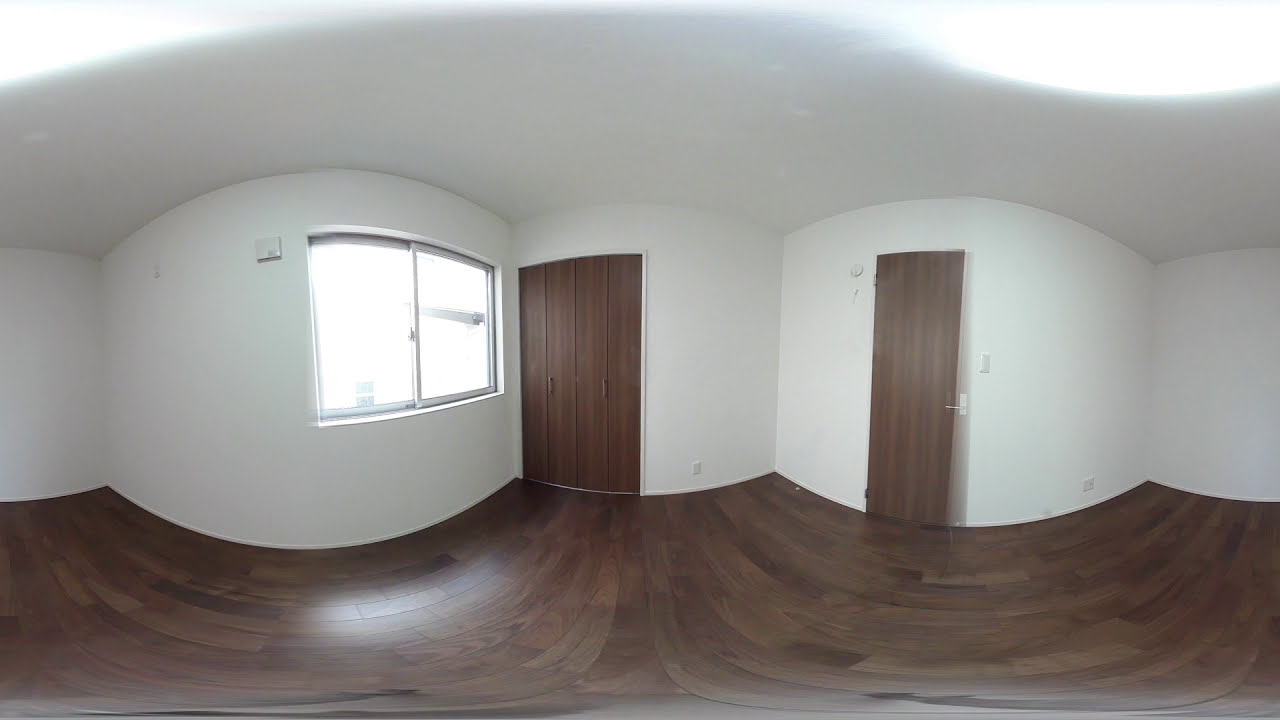The image is a distorted, panoramic view of an empty white room, taken with a 360-degree camera, giving it a stretched and curved appearance. The room features pristine white walls and ceiling, creating a bright and airy atmosphere. The floor is a dark, grainy brown hardwood, adding a rich contrast to the white surroundings.

On the left wall, there is a rectangular sliding window with a silver frame that allows ample daylight into the room. Beneath it, a plastic rectangular device, likely a smoke detector, is mounted alongside a light switch panel. The left area also features a set of brown hardwood double doors, presumably closet doors. In the center of the room, the most prominent feature is a multi-paneled door with flat, oblong silver handles. Next to it, on the right wall, is a single-paneled door with a turning handle, typically used for entering or exiting the room. Near this door, a power outlet can be seen at the bottom corner of the wall.

Incorporating all these elements, the image provides a comprehensive and detailed overview of a clean, functional indoor space with modern fixtures and efficient design.